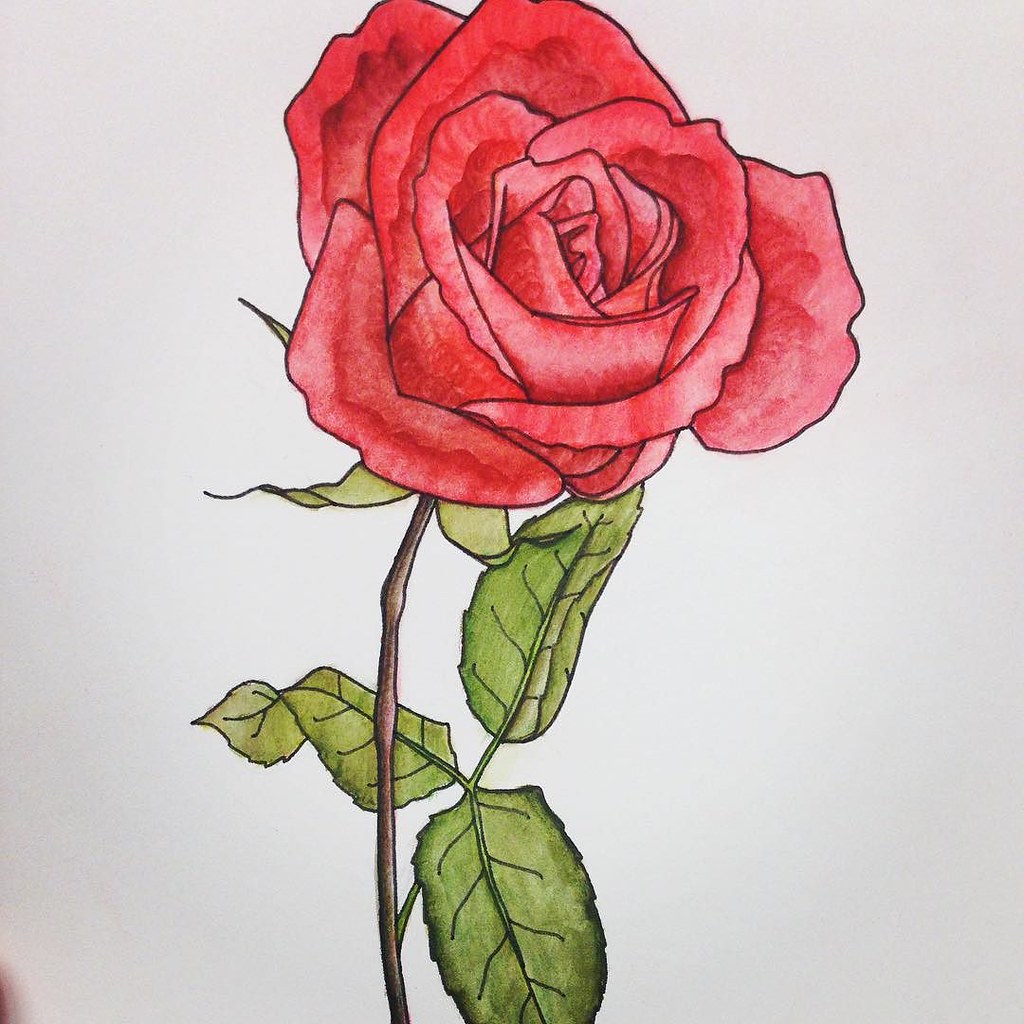The photograph captures a detailed drawing of a rose on a piece of white drawing paper. The rose features light red to pink petals outlined in black, showcasing intricate artistry. The slender brown stem extends downward, adorned with textured green leaves that display detailed edges and visible veins. The rendering does not include any thorns on the stem. In the bottom left-hand corner, part of a finger can be seen holding the paper up, suggesting the artist's presence. The skillful execution of the drawing highlights the artist's talent and attention to detail.